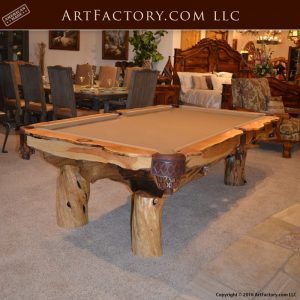The image showcases a unique and rustic-looking pool table, prominently set in what appears to be a furniture store. The pool table stands out with its legs made from stumps of trees, giving it a natural and sturdy appearance. The outer side is crafted from wood, complementing the brown felt playing field. The table features leather pockets and stands on a brown concrete floor, adding to its rugged aesthetic. In the background, a bedroom set and a dining room table are visible, reinforcing the impression of a furniture store setting. At the top of the image, "artfactory.com LLC" is clearly written across a brown bar, with an unreadable stamp next to it. The overall color palette comprises various shades of brown and tan, enhancing the rustic theme. No pool balls or cues are seen on the table, emphasizing its display condition. Additionally, there is a copyright mark in black at the bottom right corner of the image, though the name is unclear.